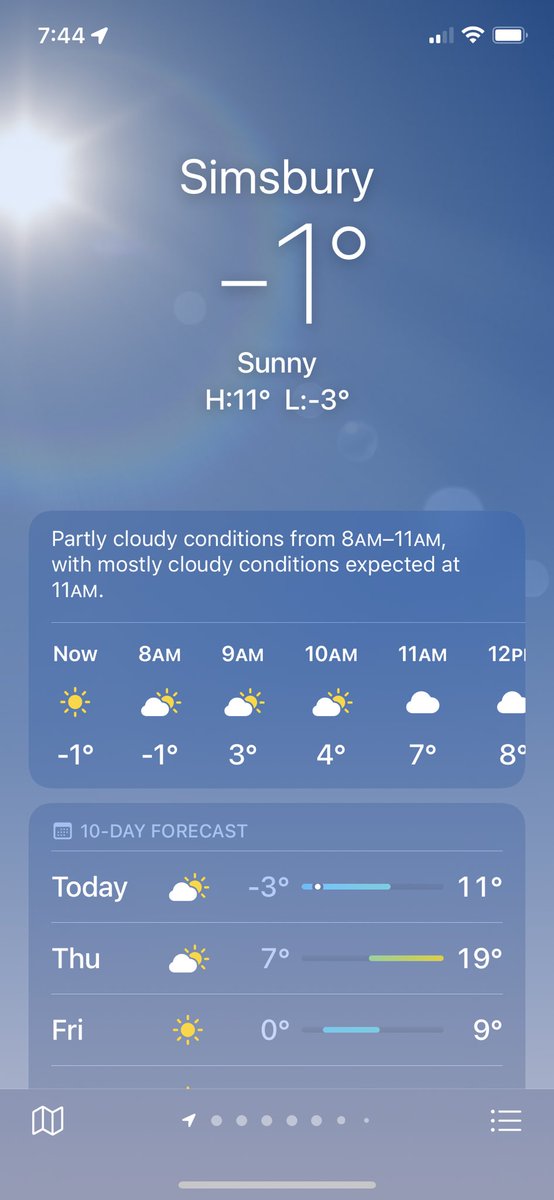Title: Detailed Weather App Screenshot

Caption: The image captures a screenshot from a mobile weather application with a blue background. Prominently featuring the sun with a rainbow halo around it in the upper right-hand and upper left-hand corners, the app indicates the current time as 7:44 AM in white text located at the top left. Next to the time, there's a small arrow button whose purpose is unclear.

On the right-hand side of the top bar, various status icons are displayed: the mobile signal strength shows two bars, Wi-Fi strength shows three bars, and a full battery icon, albeit without a percentage indicator.

Centered on the screen is the weather information for Simsbury. The current temperature is minus one degree Celsius, with a condition of "sunny." The high for the day is forecasted to be 11 degrees, with a low of minus three degrees. Below this, the app provides a brief forecast, stating that partially cloudy conditions are expected from 8 AM to 11 AM, with mostly cloudy conditions expected thereafter.

The hourly forecast beneath this section starts with 7 AM stating "sunny" at minus one degree. Subsequent hours forecast as follows:
- 8 AM: Partially cloudy, minus one degree
- 9 AM: Partially cloudy, three degrees
- 10 AM: Partially cloudy, four degrees
- 11 AM: Cloudy, seven degrees
- 12 PM: Cloudy, eight degrees

A ten-day forecast is also visible, indicating:
- Today: Partially cloudy, temperatures ranging from minus three to 11 degrees
- Monday: Partially cloudy, temperatures ranging from seven to 19 degrees
- Friday: Sunny with temperatures between zero and nine degrees

On the left side of the screen, there's a small book icon. In the middle, there are a series of dots, possibly indicating pagination or navigation options. At the lower right-hand corner, a hamburger menu icon is present, and a horizontal bar extends across a third of the screen's width just above the bottom edge, likely indicating a scroll bar or navigation bar.